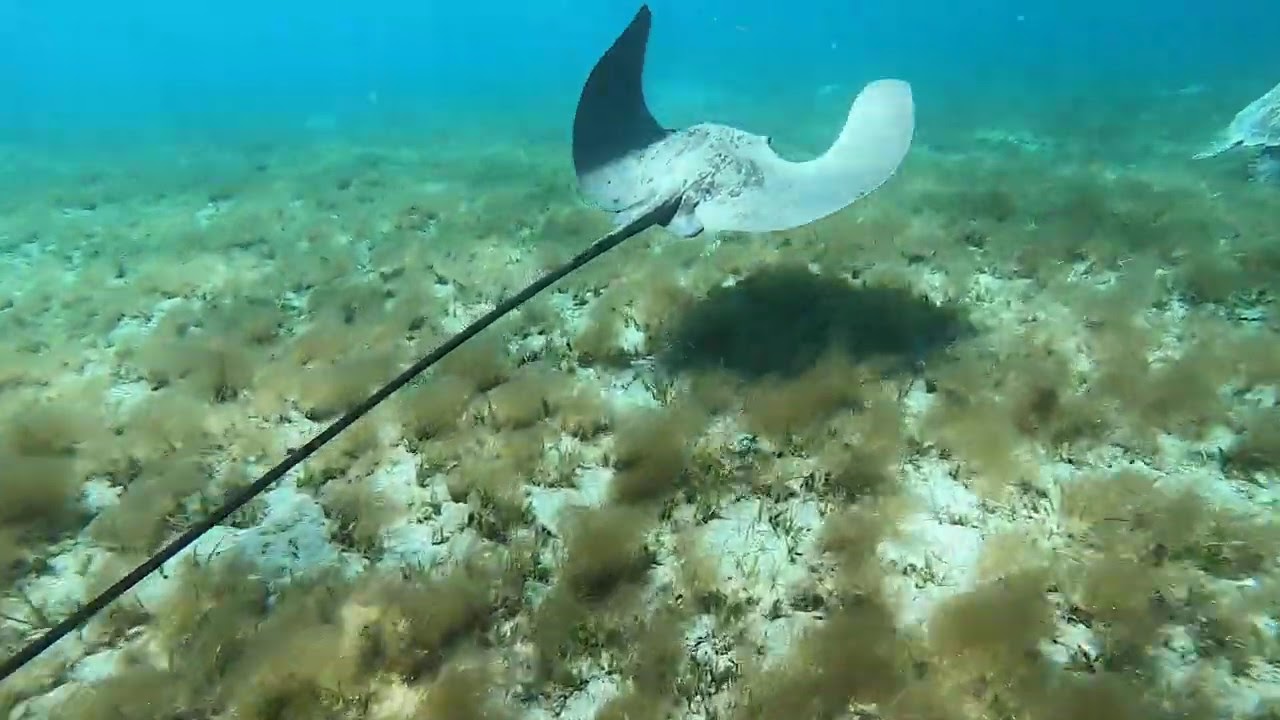The photograph captures an underwater scene featuring a stingray swimming above the sandy ocean floor. The stingray, appearing gray with its flippers or "wings" uplifted, forms a U-shape as it glides. A defining feature is its very long, thin black tail stretching from the center of the image to the bottom left corner and extending out of the frame. The sandy seabed below showcases scattered clumps of seagrass or brownish shrubs, adding texture to the scene. In the upper right corner, partially visible, is what appears to be the back left leg of a sea turtle. The water's color gradient transitions from a clear bright blue close to the stingray to a darker, murky blue in the distance, with a band of turquoise near the top fifth of the frame. The composition gives the impression that the photographer is following the stingray from behind as it navigates this vibrant underwater environment.